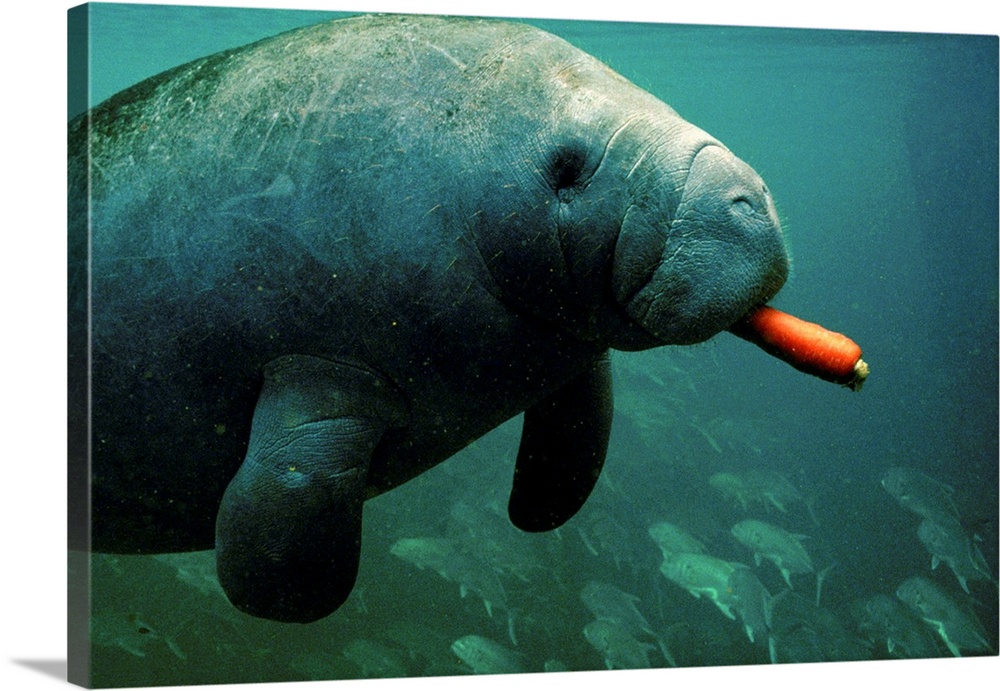The image depicts an underwater scene with a large walrus in the foreground, diagonally positioned from the left side towards the right. The walrus has a vibrant orange carrot with a green stem sticking out of its mouth, notably the only vivid color in the predominantly greenish-blue hued canvas. The walrus's eye and two of its front flippers are visible, indicating its horizontal movement. Below the walrus, a school of medium-sized, lighter-colored fish swim from the bottom right to the top left. The background includes subtle shading, particularly on the bottom left, giving depth to the scene. The entire image is presented on a canvas with visible edges, indicating it's designed as a product mock-up with a studio-like white background and some shadowing.